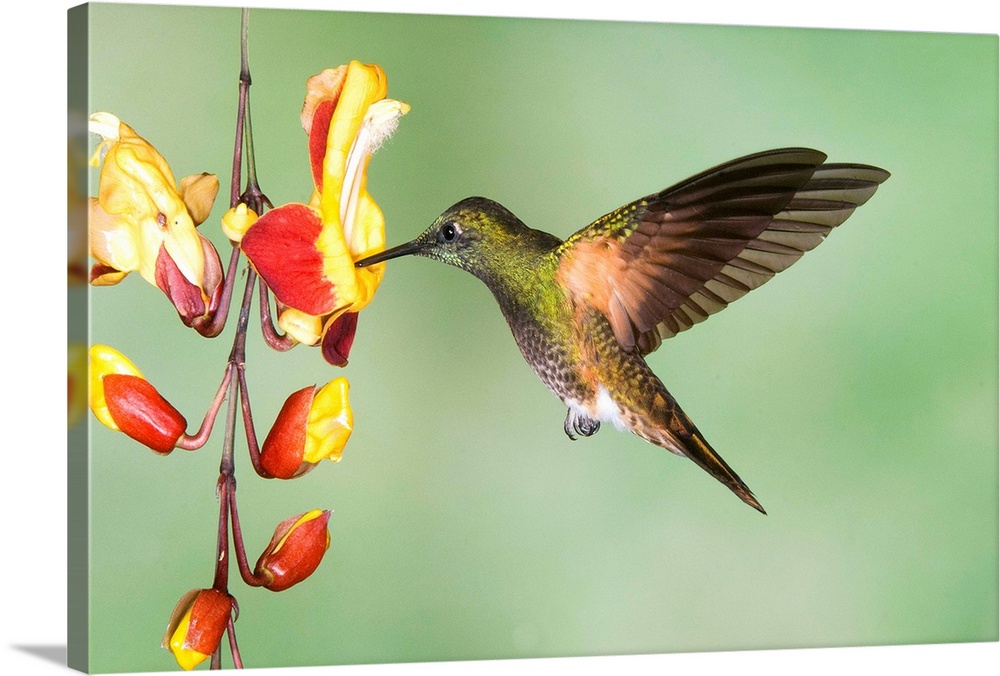The image captures a detailed view of a hummingbird in mid-flight, feeding from a honeysuckle flower. The hummingbird, positioned to the right and slightly angled, shows off its vibrant, green back and head, contrasted with a charcoal-gray chest speckled with black dots. Its tail transitions to a brown hue, while its wings, primarily dark brown with a tinge of green, appear slightly translucent. The bird's black beak is perfectly aligned with the flower, which features a plush, yellow tip surrounded by red-tipped petals. The flower itself has a long, red stem adorned with a series of unopened bulbs, creating a dynamic composition. The background is a soft blur of green and white, highlighting the hummingbird and the flower in sharp focus. The entire scene is presented on a slightly rotated rectangular prism, adding a unique 3D effect to the image.